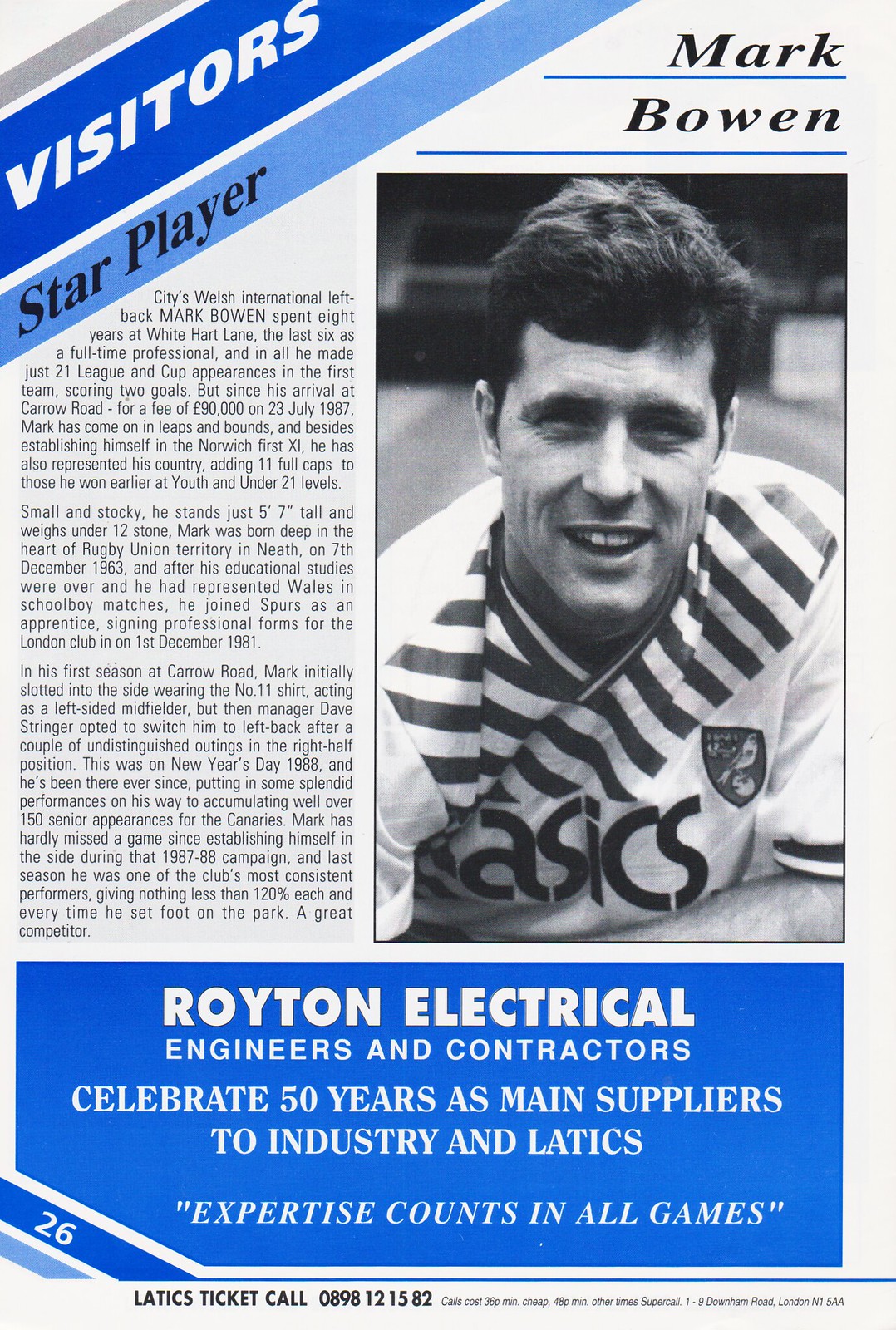This vintage football program page features a black and white photograph of Welsh international left-back, Mark Bowen, smiling at the camera. He is donning a striped ASICS jersey. The top banner of the page reads "Visitors, Star Player" with Bowen’s name prominently displayed. Mark Bowen, who spent eight years at White Hart Lane, the last six as a full-time professional, has made 21 league and cup appearances, scoring two goals. Since his £90,000 transfer to Carroll Road on July 23, 1987, Bowen has flourished, not only securing his position at the club but also earning 11 full caps for his country. Mark Bowen, born in Neath on December 7, 1963, stands at 5 feet 7 inches and weighs under 12 stone, adopting a small but stocky build. An advertisement at the bottom celebrates Royton Electrical Engineers and Contractors' 50 years as main suppliers to industry and the Lactics. Additionally, there is ticket information and a contact phone number provided.